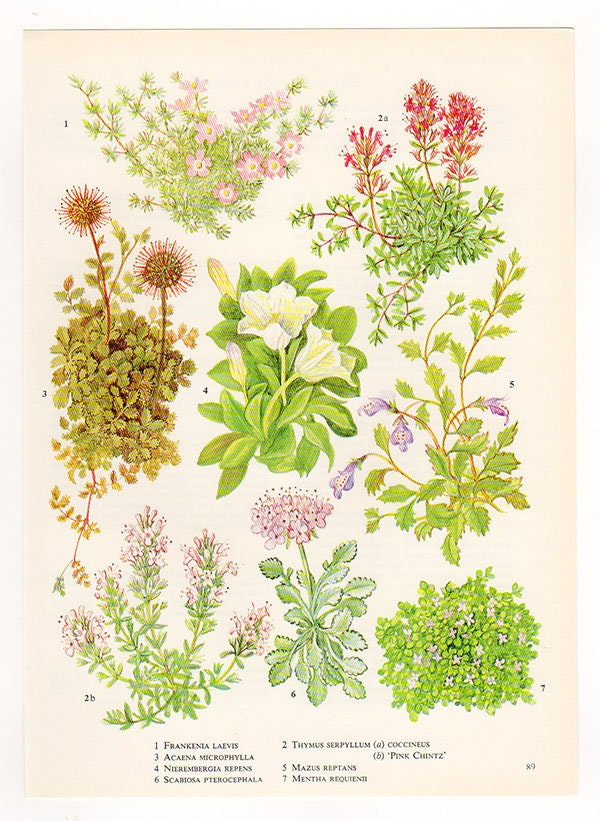This detailed image depicts a page taken from a book, characterized by its off-white, cream-colored background. It showcases seven different types of wildflowers, each meticulously drawn and colored in shades of pink, red, purple, white, and yellow. Each flower is accompanied by a small number, correlating with detailed names listed at the bottom of the page. The flowers vary in leaf shape, featuring both small and long leaves. At the bottom right of the page, we see it labeled as page 89. Among the detailed names provided, we find botanical classifications such as Frankenia lavis, Frankenia macrophylla, Nerebergia repens, Scabonia piscepolea, Thymus saraphytum, Coconus and pink chintz, Mexus Reptiles, and Menthilla requestini, written in a couple of numbered rows.